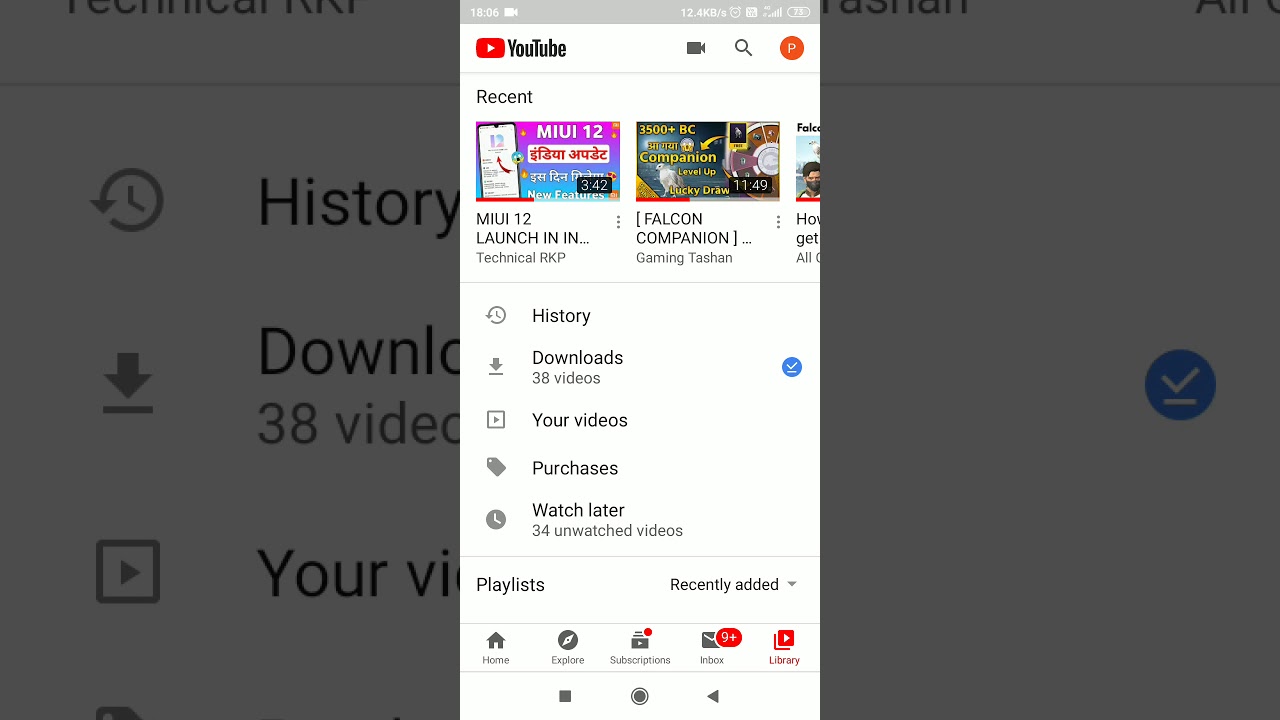In the background, a shadowed gray color creates a muted backdrop. Dominating the image is a circular arrow, almost forming a complete circle but ending in an arrowhead, symbolizing a continuous loop. Inside this arrow, the word "History" is prominently featured in black text.

Directly below this, a gray downward-pointing arrow is accompanied by a horizontal gray line. Next to this element, partial letters spell out "DOWNLO", likely indicating "Downloads". Below that, the text "38 videos" provides a numerical context.

On the image, a square encloses a gray downward arrow with the term "YourVI" nearby. Centrally positioned is a long rectangular box. At its top, a red square with a white arrow inside is adjacent to the word "YouTube". To the right of this, a small video camera icon is followed by a search bar and a red circle containing the letter "P".

Below this section, "MIUI 12 launch" is highlighted in a text box featuring pink and blue hues, with an image of a smartphone. Following this is the text "(Falcon Companion Gaming Taschen)" in parentheses.

Underneath, categories such as "History", "Downloads", "38 videos", "Your Videos", "Purchases", and "Watch Later" are listed. Additionally, there is a note of "34 unwatched videos". To the left is the heading "Playlists", while on the right is "Recently Added".